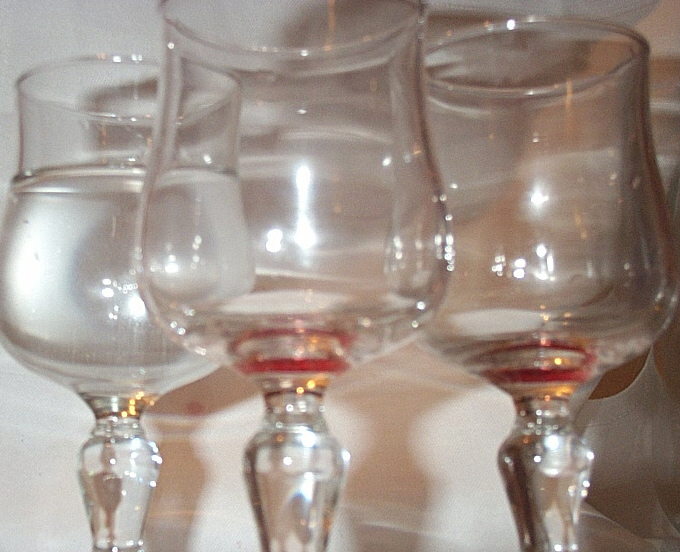This landscape-oriented image captures a close-up shot of three elegant stemware glasses, arranged side by side against a pure white background with a hint of beige and gray tones. Each glass features a smooth, slender stem leading up to the bowl, which is designed to hold wine or water, ideal for a dinner party setting. Prominently, two of the glasses in the middle and right have a vivid red outline at the junction where the bowl meets the stem, while the glass on the left lacks this red rim and is filled with a clear liquid, possibly white water. Notably, a soft, orangey glow from a light source on the right casts shadows and adds a warm reflection at the base of each glass, accentuating their shiny, smooth surfaces. The stemware is curvy and thick, making them comfortable to hold, and the image perfectly captures the delicate, crystal-clear nature of the glasses, with light playfully reflecting off their rims and stems.